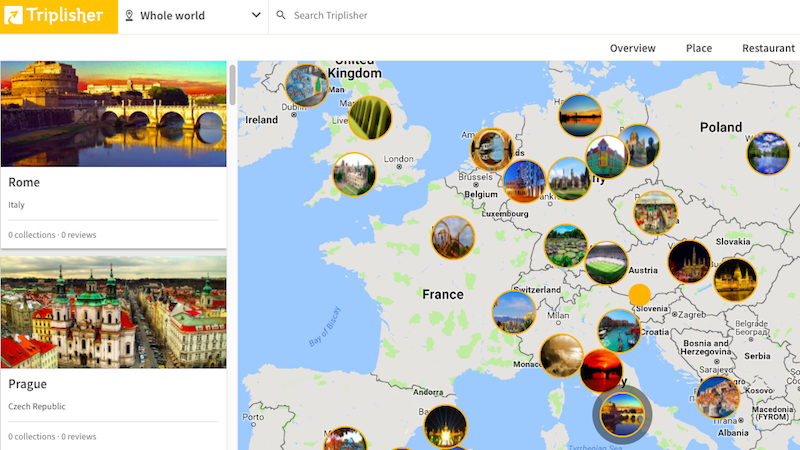Screenshot of the Triplisher app interface: 

At the top right corner, there's a distinctive yellow rectangle prominently displaying the Triplisher logo. Adjacent to the logo on its right is a drop-down menu, currently set to "Whole World". 

Dominating the central top portion of the interface is a sleek search bar, clearly labeled "Search". 

On the left side of the screen, there's a vertical scroll box designed for navigation through various locations. At the very top of this scroll box, "Rome, Italy" is listed, followed by "Prague". Users can continue scrolling to explore additional countries and cities.

The right side of the interface is largely occupied by an expansive interactive map. This map is dotted with circular icons, each featuring a photo of a notable landmark, resembling pin drops that mark different countries and their notable sights.

Above this map, towards the top right, there are three tabs labelled "Overview," "Place," and "Restaurant," allowing users to filter the displayed information accordingly. 

The entire interface rests against a clean, white background, ensuring that all interactive and visual elements stand out distinctly.